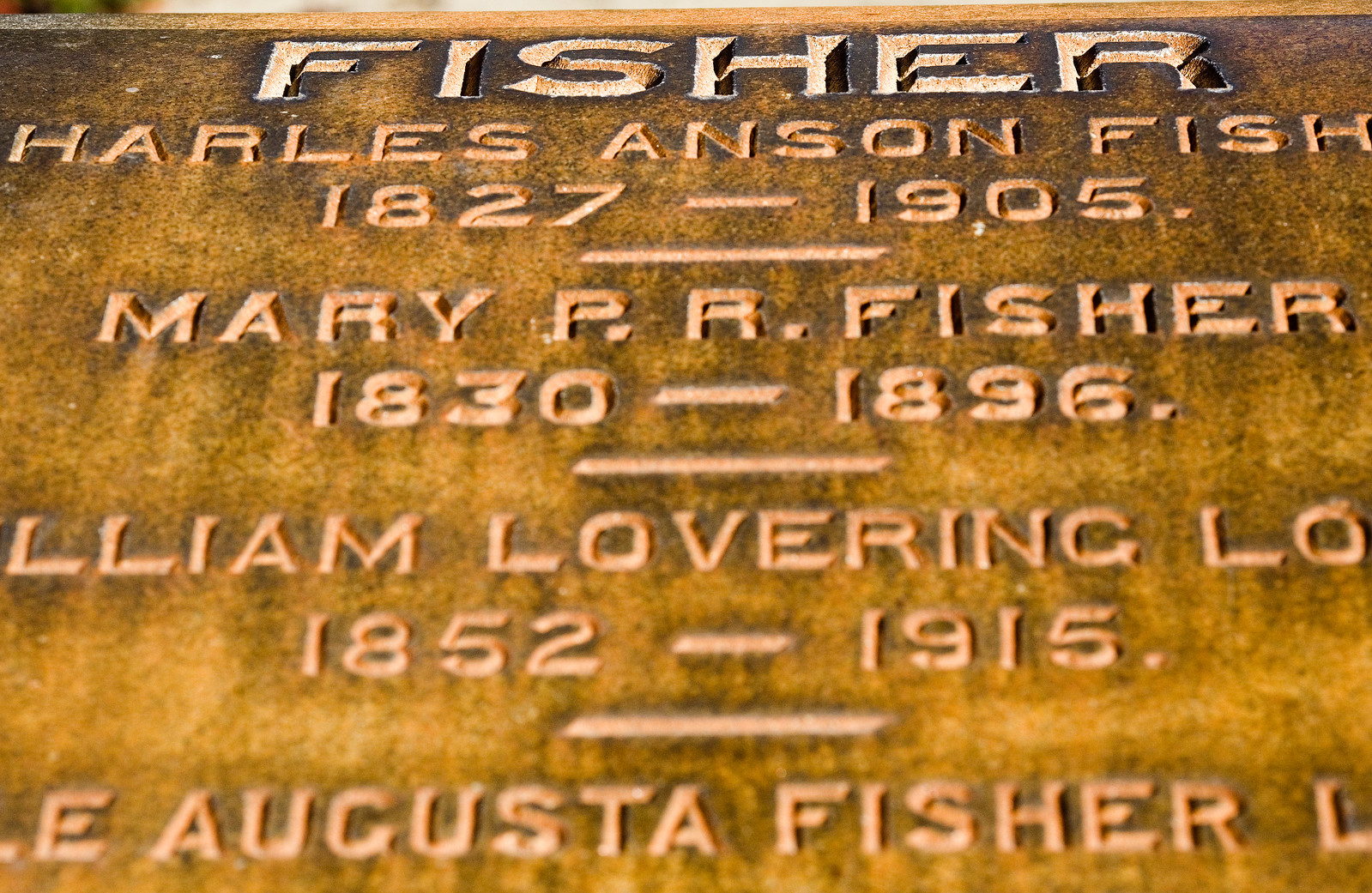This detailed engraving on a weathered, golden-yellow-brown tombstone appears to be a close-up image of a family burial plot. The headstone's surface is aged, showing signs of rust and dark bleeding from the engraved letters, giving it a rich, historical appearance. At the top, the prominent name "FISHER" is engraved in capital letters. Below it, the names of the individuals buried here are partially visible due to the close-up nature of the photograph and some damage to the stone:

- **Charles Anson Fisher (** missing the 'C'), 1827-1905 
- A faint horizontal line 
- **Mary P. R. Fisher, 1830-1896**
- Another faint horizontal line 
- **William Lovering Fisher (**missing 'W-I'), 1852-1915**
- Yet another partial listing 
- **Augusta Fisher** (without visible dates).

Each name appears followed by a period, hinting at a stylistic choice in the engraving. Despite wear and missing fragments, the headstone provides a poignant glimpse into the lives it commemorates.